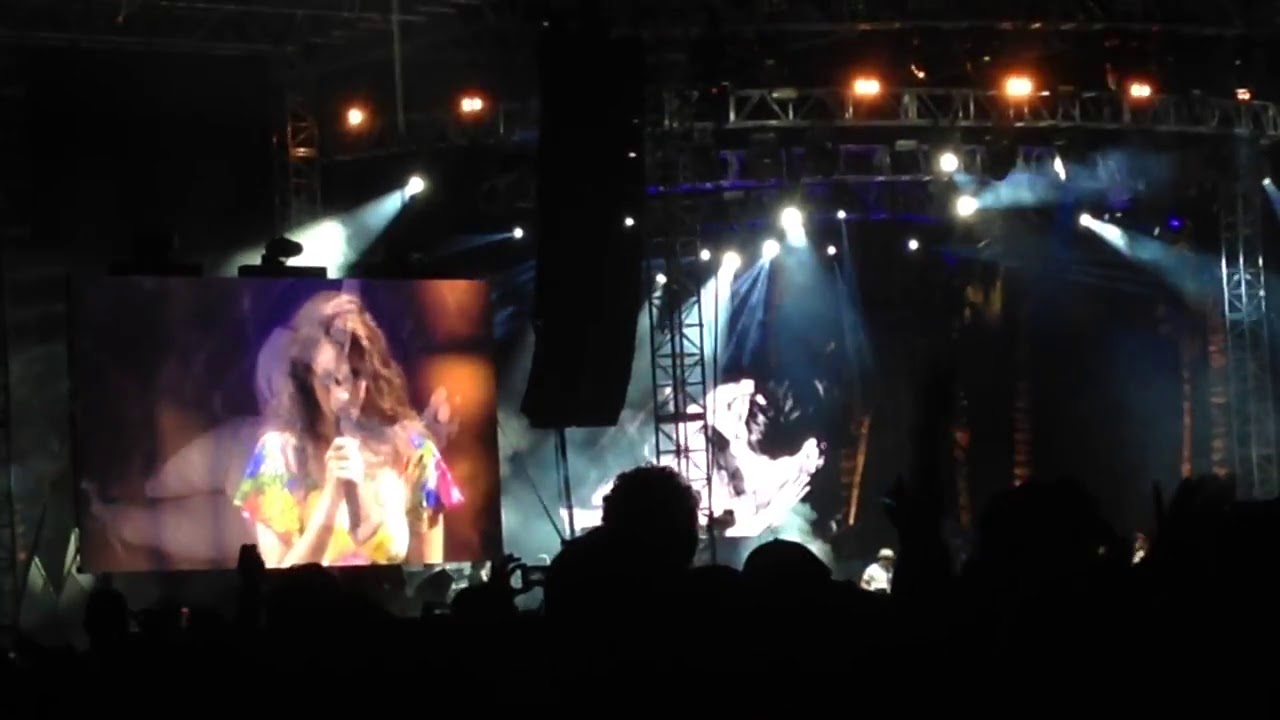In the image, we are immersed in the atmosphere of a dark concert venue. The foreground is filled with the black silhouettes of audience heads, some with arms raised, likely taking photos or videos with their cell phones. Dominating the upper portion of the image is a metallic, gray scaffolding structure adorned with sparse photographs and numerous stage lights. These lights, affixed to the bridge-like girders, glow various shades of white and yellow, cutting through the smoky air. Below the scaffolding, several spotlights cast beams in all directions, enhancing the dynamic feel of the scene.

On the left side of the image, a large square video screen captures the performance, displaying a slightly blurry but vivid image of a woman singing. She has thick, brown wavy hair and is dressed in a colorful yellow blouse, possibly tie-dye. Holding a black microphone to her mouth with her right hand, she stands out as a focal point amidst the swirling white, blue, and black hues of the stage lights. Despite the dim overall lighting, the smoke and light beams create a mesmerizing visual effect, adding to the electrifying concert ambiance.